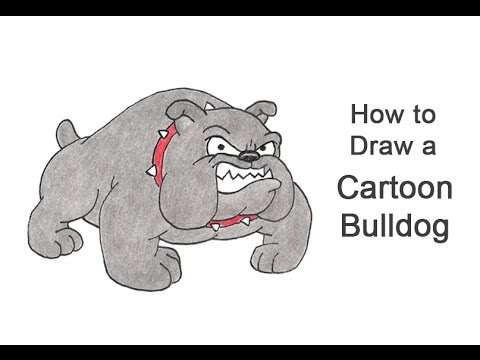This YouTube thumbnail features a detailed, colored pencil drawing of an animated, cartoon bulldog set against a simple white background. The image has thin black borders at the top and bottom, giving it a resized appearance. The text "How to Draw a Cartoon Bulldog" appears prominently on the right side, each word starting with a capital letter. On the left, the central figure is a muscular, gray bulldog with short ears, a small gray tail, and jowls hanging beside his mouth. He has a black nose, white eyes with black pupils, and bared, jagged teeth in a grimacing grin. Wearing a distinctive red spiked collar, the bulldog looks intently at the viewer. The detailed drawing only uses the colors gray, red, black, and white, and the outlines appear to be done in pen over pencil. Though the image does not show drawing steps, it's implied that it is part of a larger instructional series.